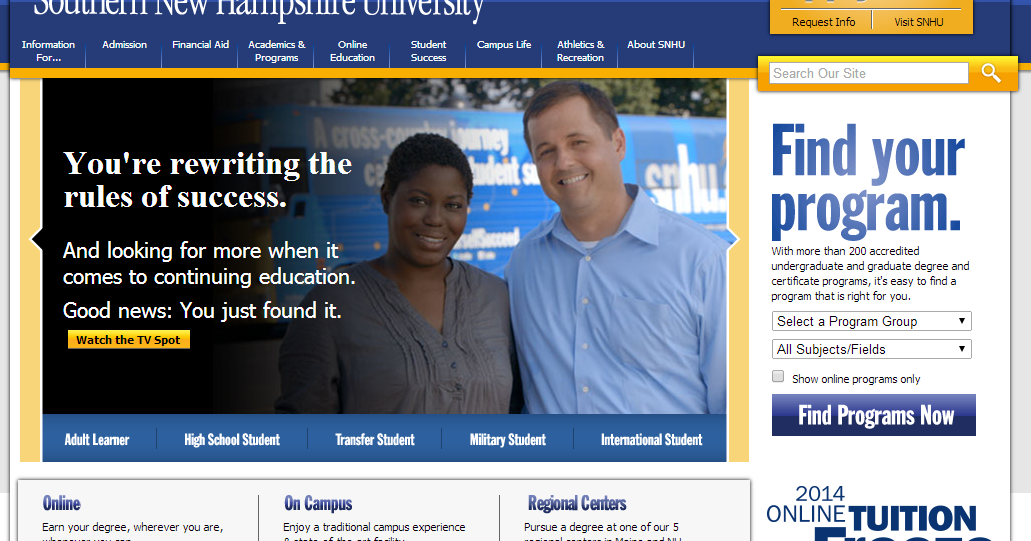Website homepage for Southern New Hampshire University (SNHU):

The top section of the website is partially obscured, displaying only the lower half of the university's name, "Southern New Hampshire University," against a blue background. The navigation menu provides links to essential areas: Admissions, Financial Aid, Academics & Programs, Online Education, Student Success, Campus Life, Athletics & Recreation, and About SNHU. 

On the upper right corner, there are options to "Request Info" and "Visit SNHU," followed by an orange line that stretches horizontally across the page. To the right of this line, there's a search bar labeled "Search our site."

Below the navigation, a prominent photograph features a smiling white man standing beside a black woman. Accompanying this image is a message in white text: "You're rewriting the rules of success and looking for more when it comes to continuing education. Good news, you just found it." Beneath this motivational message, a bright orange button invites visitors to "Watch the TV Spot."

To the right of the image, text encourages visitors to "Find your program" with an array of over 200 accredited undergraduate and graduate degrees, along with certified programs and certificates. A dropdown menu labeled "Select Program Group" and another labeled "All Subjects/Fields" offer filtering options. Visitors can also select a checkbox to "Show Online Programs Only," and a button labeled "Find Programs Now" completes the search tools.